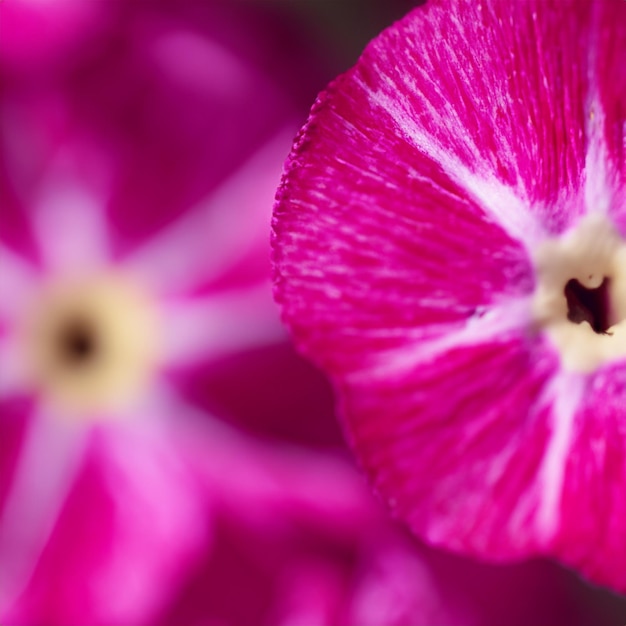This is an extremely close-up, macro photograph featuring two vibrant fuchsia flowers with intricate detailing. The primary focus is on a flower on the right side of the image, showcasing its deep pinkish-purple petals with delicate cream-colored centers that fade into thin white streaks. The petals are frilly and exude a sense of delicacy, creating a striking visual contrast against the richly colored fuchsia. The flower on the left side of the photograph is the same type but appears larger and is out of focus, serving as a blurred background. Despite being out of focus, it shares the same fuchsia hue with white and cream striping and hints of a light yellow center. The flowers' intricate patterns and vibrant colors are reminiscent of those you might encounter in a meticulously maintained city garden.